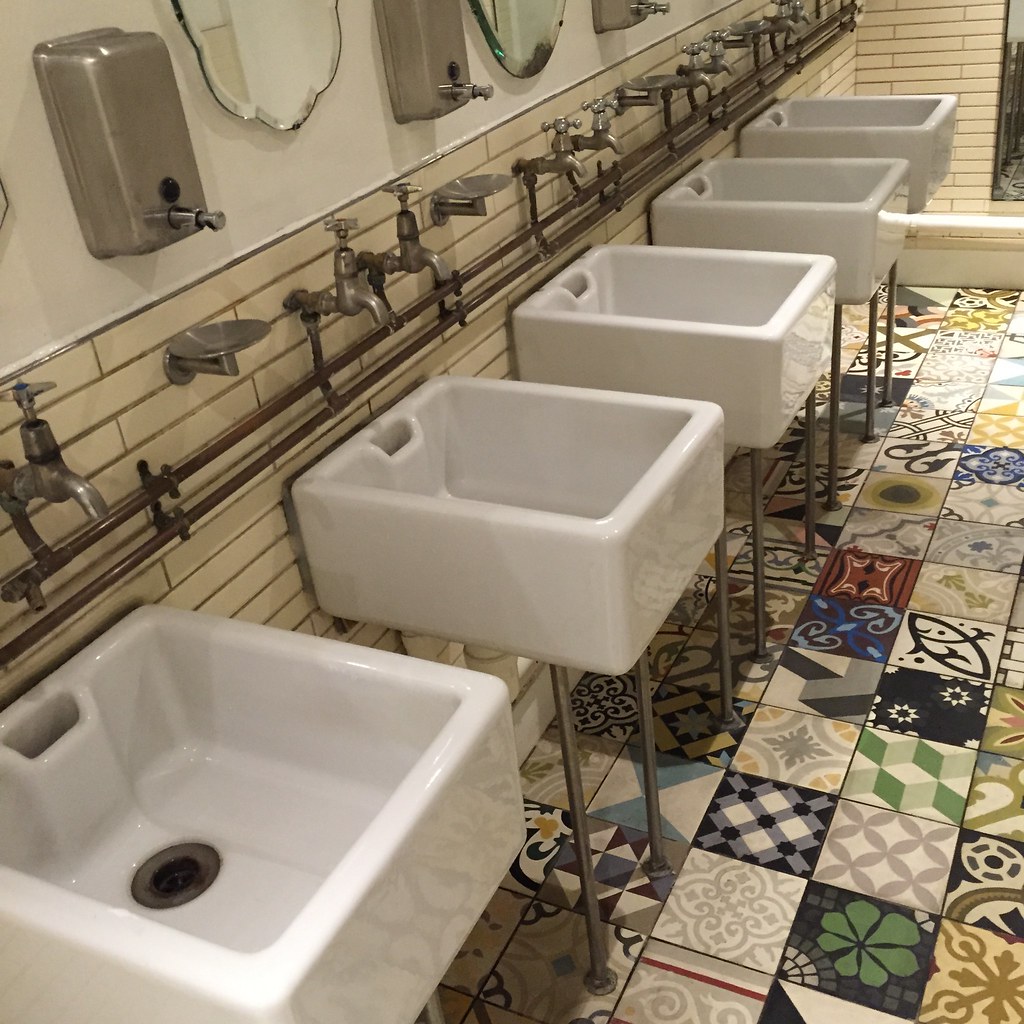The image depicts a public bathroom featuring a row of five white ceramic sinks, each supported by two chrome steel posts at the front and mounted to a wall adorned with white subway tiles. These square-shaped, white porcelain sinks are equipped with two silver spigot faucets, and old-style washer handles are visible above each sink. A continuous line of metal feeder manifolds runs along the wall, indicating the water supply to the faucets. Above the sinks, positioned on a plain white drywall, are three rectangular, metal soap dispensers with catch trays below them, flanked by small, oval mirrors with scalloped edges that lend an antique charm to the space. The floor is strikingly vibrant, featuring a patchwork of linoleum tiles in an array of colors and intricate geometric patterns. Each tile is distinct, incorporating hues of green, black, blue, yellow, and gold, resulting in a visually eclectic and chaotic design. The far wall includes a partial glimpse of a wall mirror, adding to the room's utilitarian yet distinctive aesthetic.